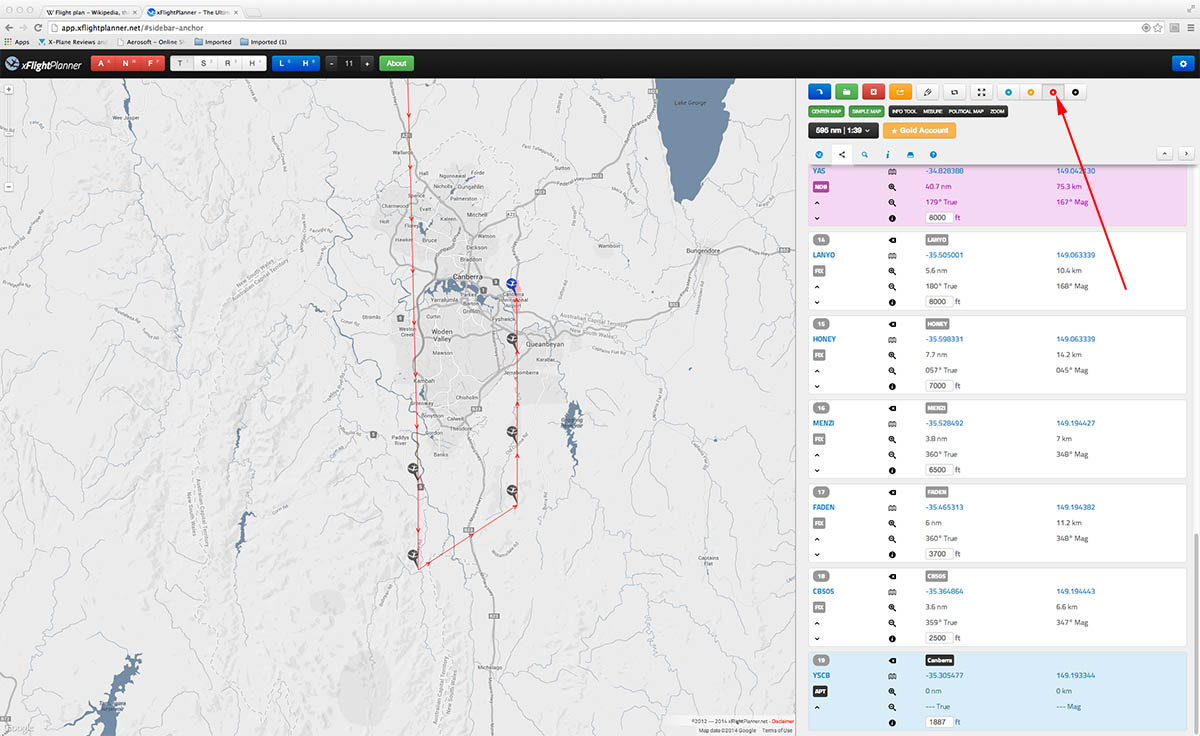The image displays the X-Flight Planner website, specifically at the URL x-flightplanner.net. The browser shows two tabs open to the same URL. Prominently featured is the X-Flight Planner interface, which appears to be a comprehensive tool for flight planning. The interface includes a detailed button panel with various labeled buttons: "A°", "N°", "F°", "T1", "S1", "A1", "H1", "L1", "H1", and "11" with a dropdown menu, along with an "About" section.

Central to the interface is a large, interactive map, flanked by an extensive data panel on the right side. This data panel includes seven horizontally extended rectangles and numerous buttons. A conspicuous red arrow points to a highlighted button, marked with a red circle, suggesting it plays a critical role, possibly in a training context. The arrow seems to have been added through photo editing software, underscoring the button's importance. This setup implies the website's use in a flight training scenario, likely for small aircraft pilots. The overall design and specific annotations suggest comprehensive flight planning and instructional purposes.